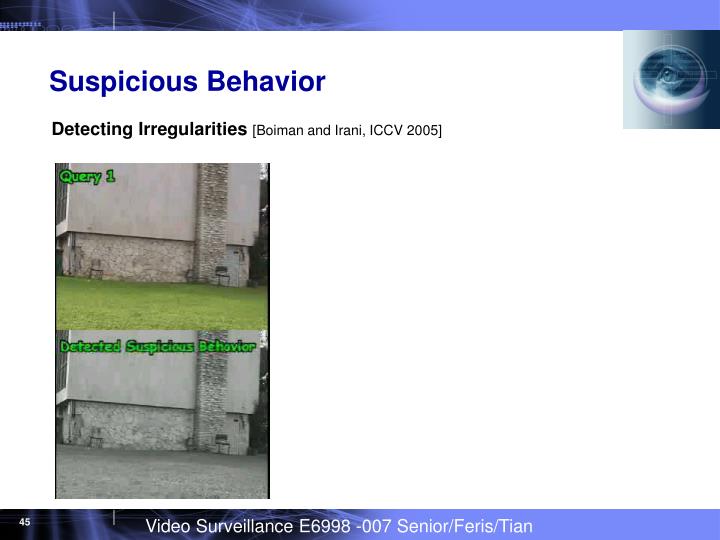The image is a full-color digital slide with a predominant white background. It features blue bands at the top and bottom, embellished with light blue decorations. In the upper right-hand corner, there is a logo of an eye within a blue square. At the top of the slide, bold blue text reads "Suspicious Behavior," followed by black text stating "Detecting Irregularities, Boyman and Irani, ICCV 2005."

On the left side of the slide, there are two photographs of the same stone building with a chimney on its right-hand side. The upper photograph is in color and labeled "Query 1," showing a green lawn in front of the building. The lower photograph is in black and white, displaying a gray lawn. In this photo, green text highlights "Detected Suspicious Behavior." Both images seem to be related to video surveillance, indicated by the text "Video Surveillance E6998-007 Senior/Ferris/Tien" at the bottom of the slide.